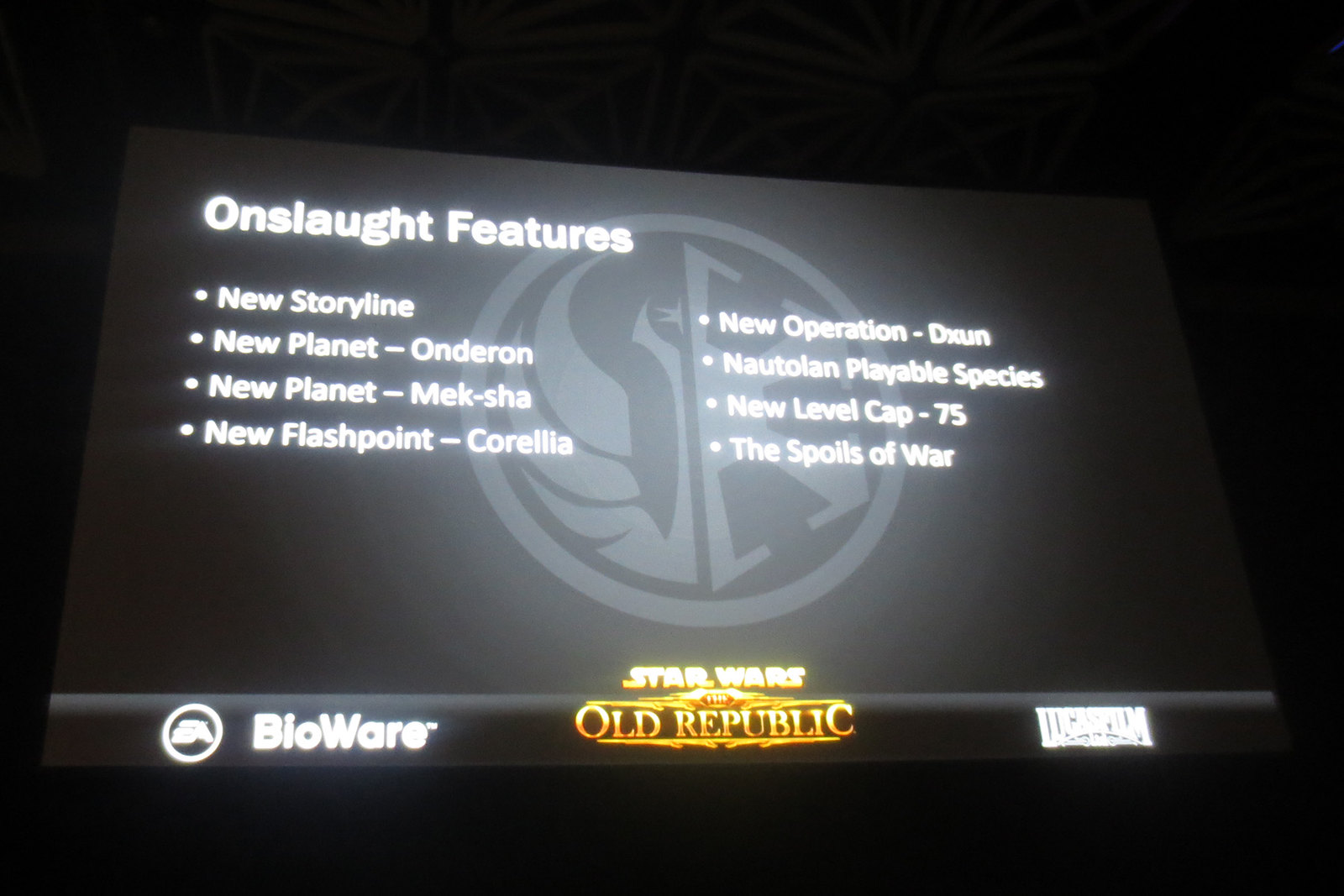The image depicts a dimly lit room featuring a large projector screen displaying promotional material for a video game, likely associated with a streaming service named Onslaught. The screen is filled with white text, with the key title "Onslaught Features" prominently displayed in the top left corner. Beneath this title, there are two columns of bullet points highlighting several new features. 

The left column lists:
- New Storyline
- New Planet: Onderon
- New Planet: Meksha
- New Flashpoint: Corellia

The right column highlights:
- New Operation: Dxun
- Nautolan Playable Species
- New Level Cap: 75
- Spoils of War

At the bottom, a black banner runs across the screen. On the left side of this banner, it reads "EA BioWare," while in the center, "Star Wars: The Old Republic" is written in golden-yellow text with a faint yellow glow. To the right, "Lucasfilm" is also visible in white text. The backdrop of the image features a dark background with a light gray circle and abstract shapes, providing a subtle contrast to the text.